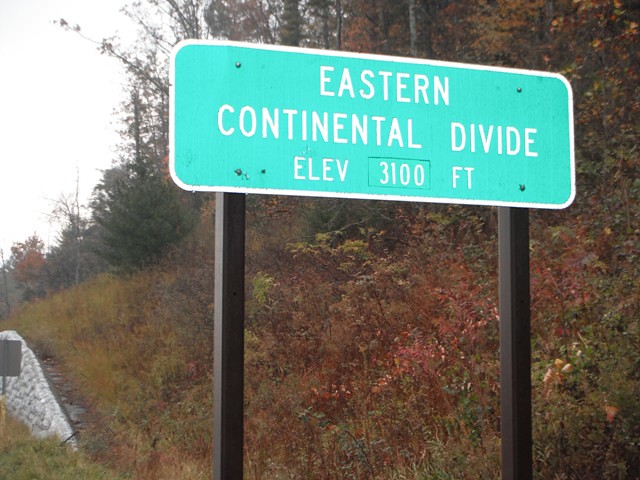This photograph captures a roadside sign that proudly announces the location of the "Eastern Continental Divide" at an elevation of 3,100 feet. The sign itself is a striking combination of green and white, prominently displayed on sturdy, vertical black posts. Behind the sign, a diverse landscape unfolds, featuring dense brush and a variety of trees alongside a gently sloping hillside. Adding an element of rustic charm to the scene, a slightly arched stone retaining wall, situated in the lower left-hand corner, provides structural support to the hillside. The overall palette of the image includes lush greens, somber blacks, pristine whites, and hints of earthy rust, creating a visually rich and detailed portrayal of this geographical marker.